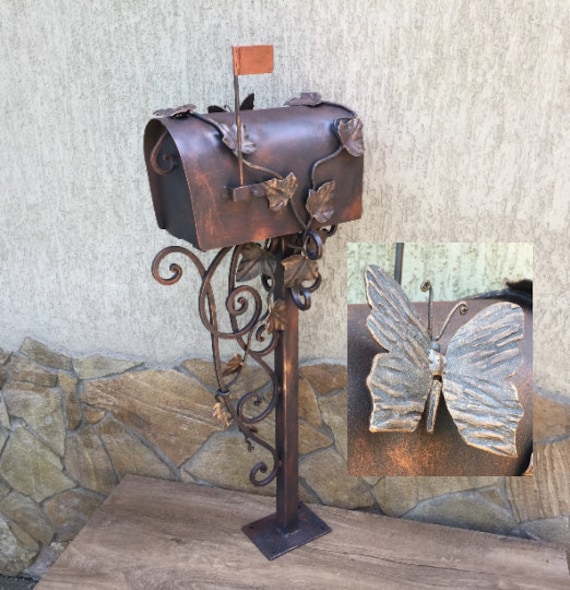The image showcases a beautifully detailed mailbox, likely made of bronze, prominently positioned at the center of the picture. The mailbox is mounted on a flat, square stand that seems to be part of a wooden bench. Intricately designed to resemble vines and leaves, the bronze structure features finely detailed foliage, with some leaves exhibiting a unique square shape. A bronze flag, indicating outgoing mail, stands upright on the side of the mailbox. Adjacent to it, a bronze butterfly perches with exquisite detailing, including curly antennae and textured wing patterns. The background presents a layered aesthetic: the lower portion is composed of a tan, gray, and brown cobblestone wall, while the upper part comprises a beige stone wall. A close-up inset at the bottom right highlights the butterfly’s intricate craftsmanship even further.